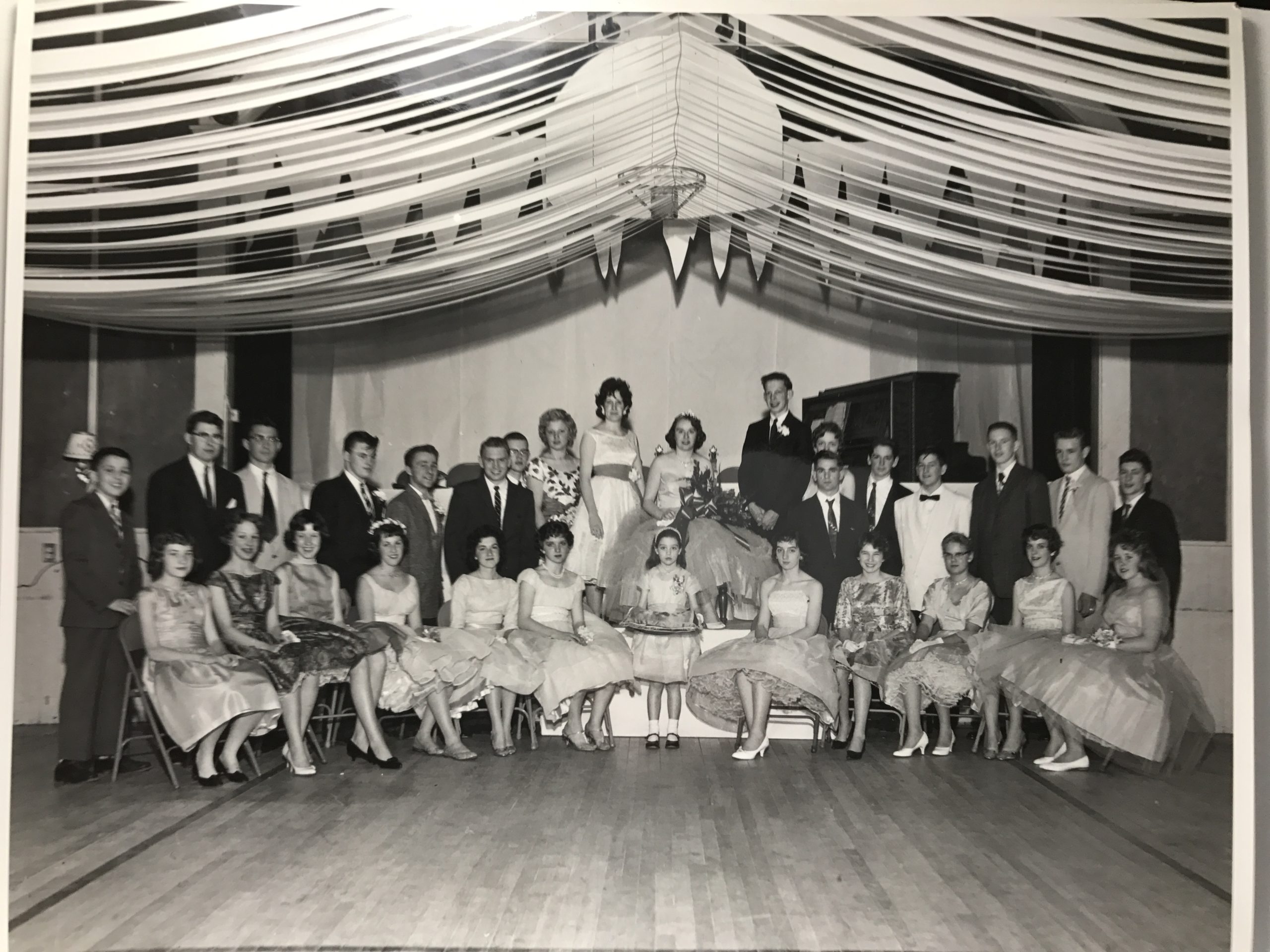This vintage black and white photograph, with a sepia tone, captures a formal event held in a large hall, possibly a school basketball court, which features a wooden floor and is decorated with ceiling canopies and other elegant designs. The group photo is composed of rows of professionally dressed individuals. In the foreground, a number of women, adorned in beautiful skirts, dresses, and gowns, are seated. Each woman in the chairs is accompanied by a man standing behind her, dressed in suits, suggesting a formal occasion such as a wedding or a school dance. At the center front, a small girl stands, adding a touch of innocence to the scene. Behind the seated women and the standing men, at the center, a lady is seated in a larger chair next to the groom, who is wearing a black suit. This ceremonious ambiance, coupled with the careful arrangement of the participants, hints at a significant celebration, possibly a wedding or an award ceremony, attended by young adults or students.